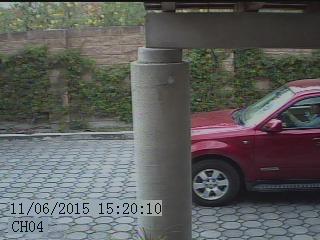The image appears to be a security camera feed taken outdoors, possibly from a driveway or a similar tiled gray surface area. Dominating the right-hand side of the image is a red SUV, of which only the front half and the side from the passenger door to the front are visible. Inside the vehicle, the side of a person's body can be seen. A prominent cement pillar with a rectangular base is located towards the center of the image, partially covering what seems to be an awning. In the background, there's a tan-colored brick wall adorned with green ivy or vines, along with trees and shrubbery. The bottom left corner of the image shows a timestamp reading 11/06/2015 15:20:10 CH04.